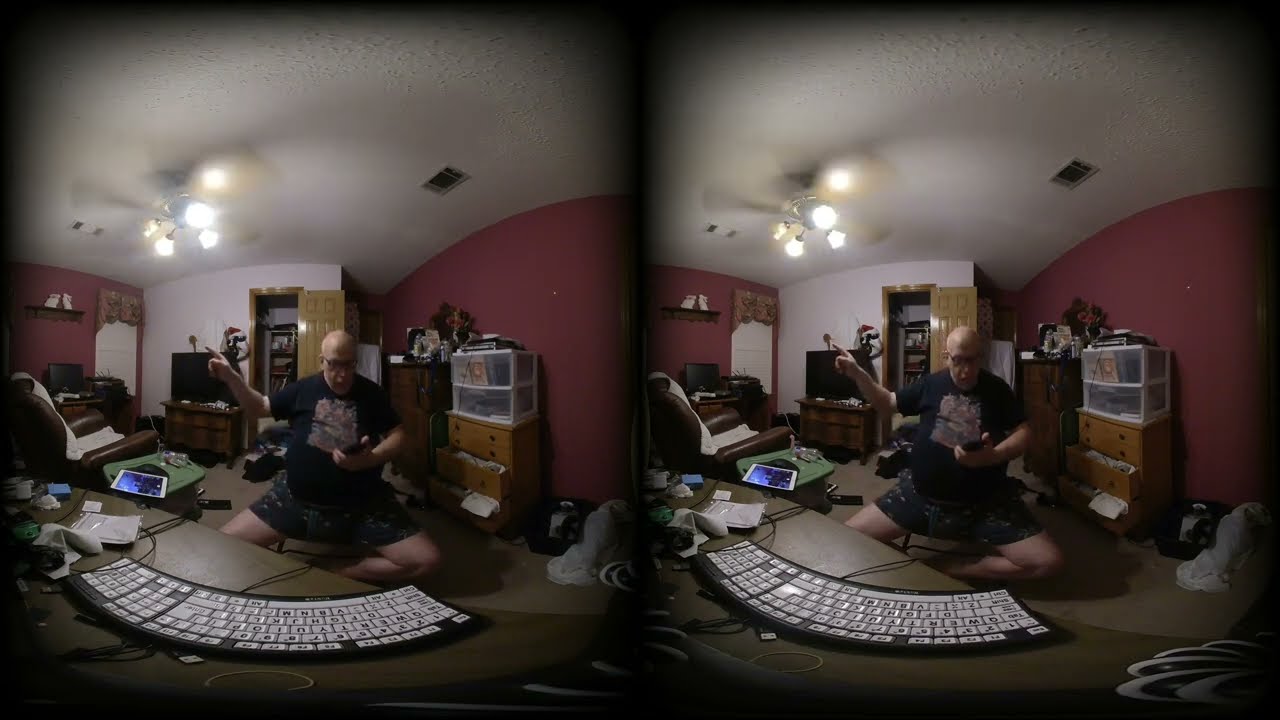In this indoor photo, arranged as two nearly identical images set side-by-side, we observe a single scene depicted twice. The focal point is a bald man wearing glasses, a dark T-shirt with lettering, and patterned dark shorts, seated on a low bench. He is facing forward, holding an unidentified object in his left hand and pointing with his right forefinger. The photographs capture a detailed view of his cluttered living space decorated with burgundy walls and various pieces of furniture and equipment.

Behind the man, a white-walled area features a door, possibly leading to a closet, and a brown recliner to his left. To his right is a set of jammed drawers with papers sticking out, topped by a small white cabinet. Further right is another cabinet filled with miscellaneous items. In front of him, a semicircular counter curves around, crowded with electronic devices and a board covered in white writing, which might be a large keyboard or some kind of control panel. The background also suggests the presence of a potential musical instrument, possibly a piano or organ, and a mixture of technology and storage spaces.

The man's gesture and the cluttered yet organized array around him suggest he is absorbed in a technical or electronic project. The overall ambiance of the space blends functional disarray with an insightful peek into his focused activity.